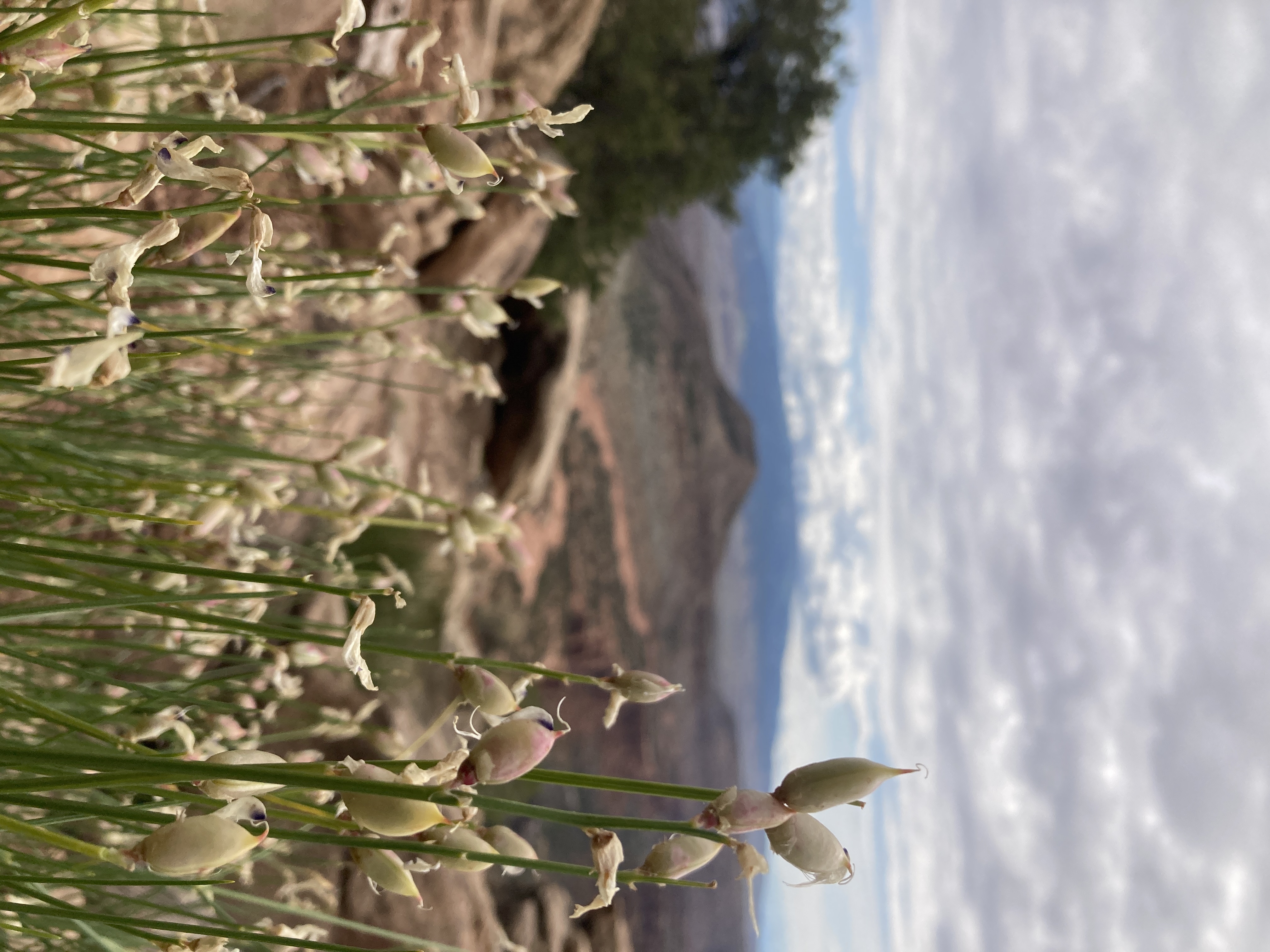The sideways color photograph, tilted to the left in landscape orientation, captures an arid but scenic landscape under a very cloudy sky. The dominant background features gray clouds looming over bluish distant mountains and closer, greener hills. In the immediate foreground, an untouched conifer stands prominently, while a wild grain, characterized by its green stems, slender leaves, and seeds, is in sharp focus. Although some flowers are present, their white petals have mostly wilted, leaving behind capsule-like bulbs. The overall scene evokes a semi-desert feel, reminiscent of locations such as Arizona or Idaho, presenting a rugged and dry environment punctuated by resilient vegetation.